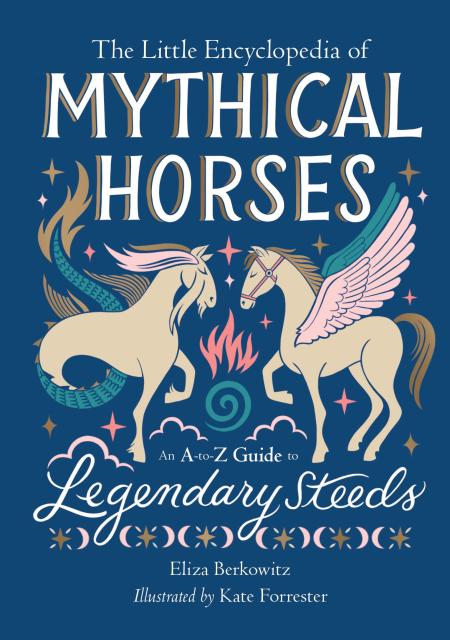The cover of the book titled "The Little Encyclopedia of Mythical Horses: An A to Z Guide to Legendary Steeds" by Elizabeth Berkowski, illustrated by Katie Forrester, features a striking and imaginative design on a dark blue background. The title is displayed prominently in large, white block letters with a delicate light gold background accentuating the text. At the top, smaller white print reads "The Little Encyclopedia of," and below, also in white, the subtitle "An A to Z Guide to Legendary Steeds" is written in a cursive font.

Central to the cover is a detailed illustration of two mythical, horse-like creatures. On the right-hand side stands a majestic pegasus, its body a light cream color with a tan mane and tail. This pegasus is adorned with a pink bridle and boasts two large wings: the nearer wing is pale pink, while the wing behind is light blue. Opposite the pegasus, on the left-hand side, is a fantastical creature with the head and two front legs of a horse, but with the serpent-like tail of a mermaid. This hybrid creature shares the pegasus's cream-colored body. It has a pink and brown mane extending from underneath its ears, a tuft of fur beneath its eye, and small chin whiskers. The serpent tail is light greenish-blue, covered in scales, and ends in a light brown, almost gold, fur-tipped fin.

This cover seamlessly combines these enchanting elements, inviting readers into a world where mythical horses reign supreme.